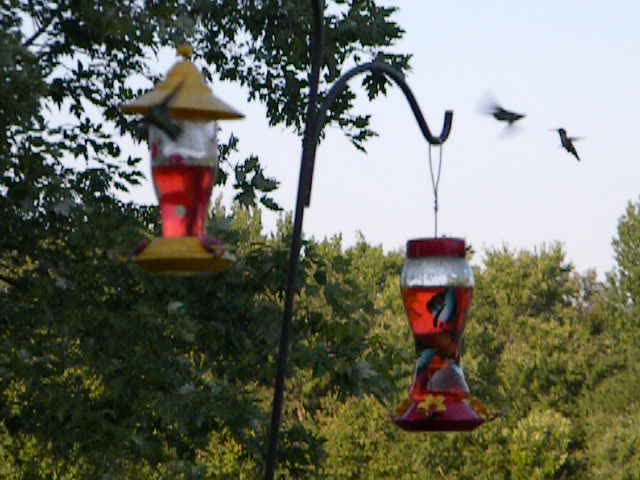In this digital outdoor photograph, we see a bright, clear sky with bluish white hues, offset by lush green foliage of varying tree sizes in the background. Prominently featured in the center is a black iron shepherd’s hook pole, splitting into two swirl hooks, each adorned with a different bird feeder. To the left hangs a unique cylindrical bird feeder with a yellow top and bottom, resembling a straw hat, and a clear middle section filled with red nectar. On the right, there is a red, cylindrical feeder with intricate designs and a transparent section, also containing red nectar. High in the upper right corner of the image, two hummingbirds are captured in mid-flight, their wings a blur due to their rapid motion. One of the birds appears to be perched on the yellow feeder while the other hovers nearby, adding a vibrant, dynamic element to the serene composition.